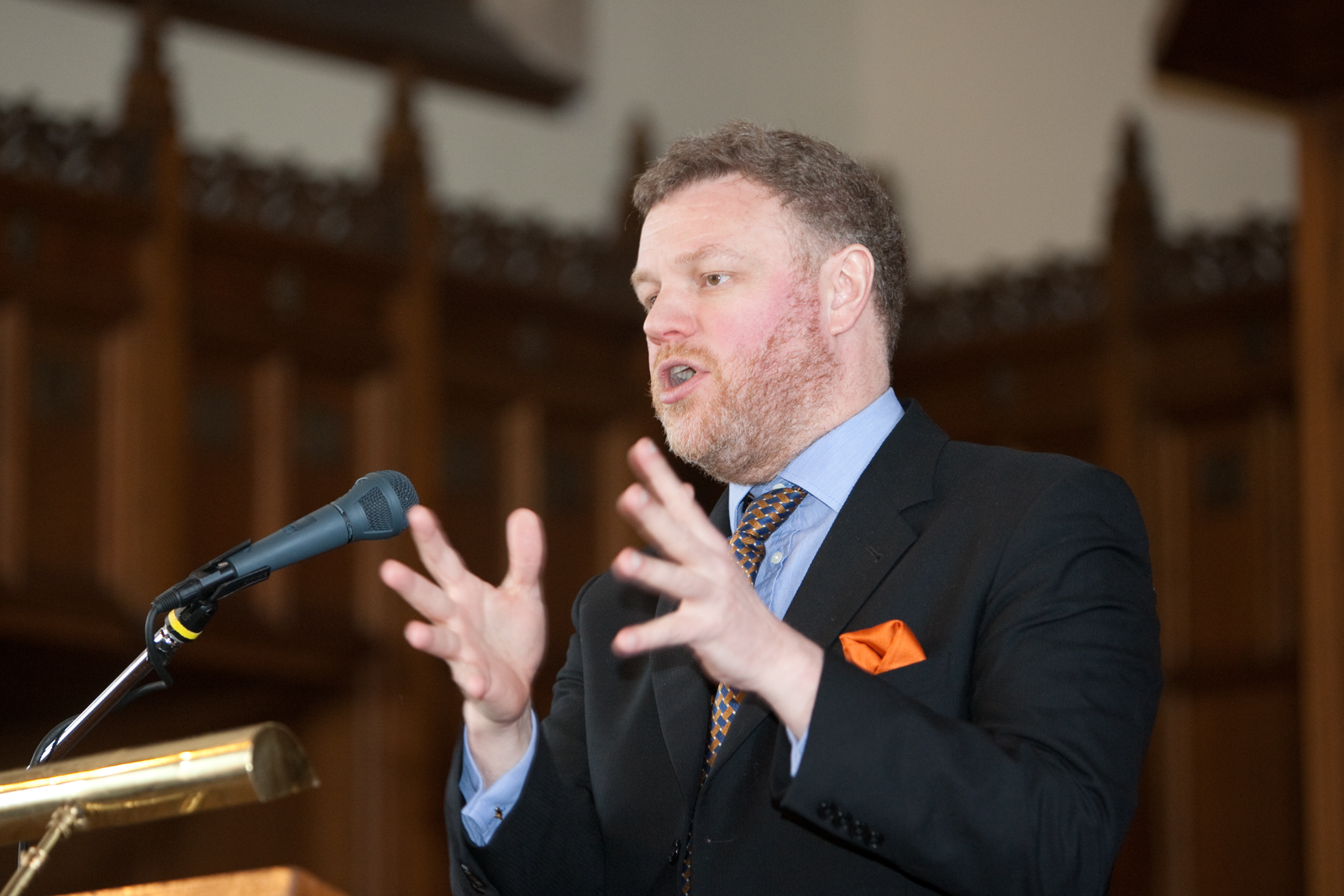This photograph captures a man, likely a politician, standing behind a partially visible podium from a slightly side view, delivering a speech. The podium features a notable gold-tinted cylindrical lamp to the bottom left and a blackish-gray microphone with a silver holder aimed towards the speaker. The man, who appears to have white skin and brown hair with some graying, is dressed in a dark suit, a light blue collared shirt, and a blue and gold alternating tie. Completing his attire, he has an orange handkerchief tucked into his breast pocket. With his hands raised in front, open-palmed, and his mouth slightly open, he is actively engaging his audience. The blurred background suggests the setting might be an ornate courthouse or castle, characterized by brown wooden walls with intricate architectural details.